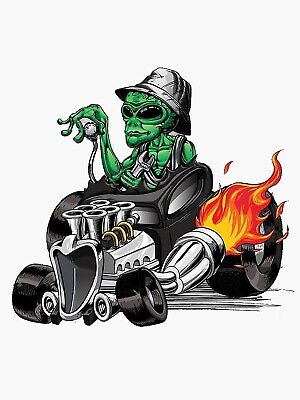This image is a highly detailed, cartoon-like drawing of a green, reptilian alien riding in a stylized hot-rod vehicle. The background is a very dark, almost clear shade, emphasizing the main subject. The alien, with its distinct green skin, has a typical extraterrestrial appearance featuring black oval eyes, a tiny slit for a mouth, and a large forehead partially obscured by a gray, creased fisher hat. It's dressed in a gray tank top, adding to its quirky appearance.

The vehicle itself is a black, flat motor car with significantly exaggerated proportions, reminiscent of a monster truck. It features two small front tires and two large back tires, with one clearly visible and another presumably obscured by the angle. The car’s design includes a prominent, silver engine in the front, equipped with six vertical tubes, emitting vibrant yellow and red flames from an exhaust in the center of the vehicle.

The alien's right hand delicately grips a silver gear shift, while its left hand holds a silver wrench. The car casts a long, horizontal shadow beneath it, further accentuating its low-slung, hot-rod style. The drawing's playful, tattoo-like style gives the overall image a vivid, dynamic, and whimsically surreal quality.